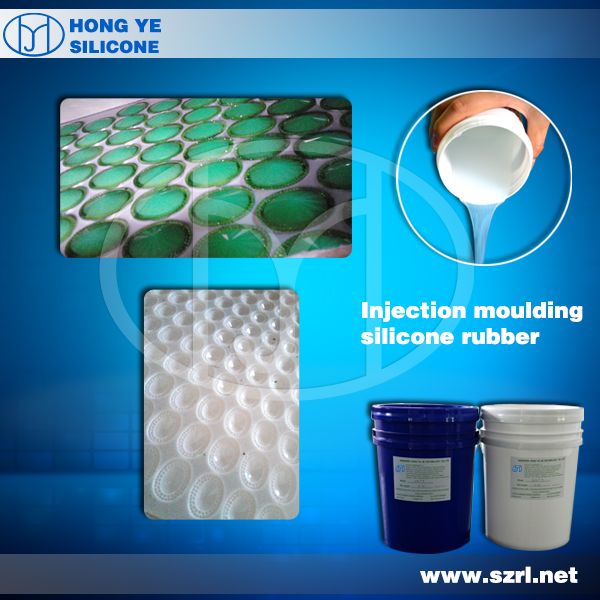The image is a promotional poster for Hongye Silicone, specializing in injection molding silicone rubber. It features a prominent logo in blue at the top-left corner, accompanied by the company name. The background is primarily blue with several distinct graphics. In the top-right corner, a hand is pouring a clear liquid from a white jar into a white circle. Below, to the bottom-right, the website www.SZRL.net is displayed alongside two buckets, one blue and one white. The top-left graphic depicts green silicone circles, while the bottom-left showcases clear circles. Overall, the image combines these elements to emphasize the various products and the company's identity.